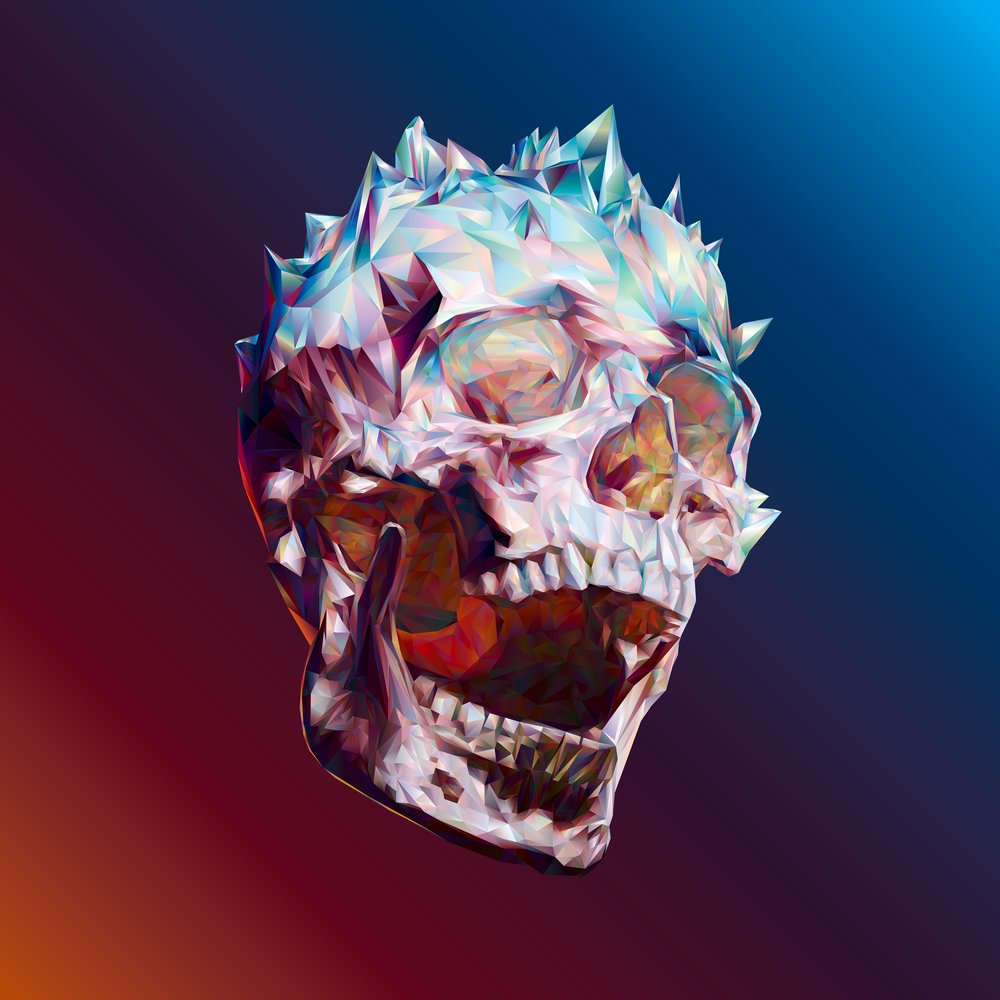This image showcases a highly detailed and vividly colored artistic rendering of a human skull. The striking skull is positioned perfectly centered within a square frame. The skull’s mouth is open, revealing all its teeth. The skeletal structure, devoid of any flesh, has hollow eye sockets and a large nose cavity, giving it a haunting appearance. The skull is adorned with jagged, diamond-shaped spikes that rise sharply from the top and back of the head, primarily in hues of light blue, pink, and yellow. The spikes form a distinct and prominent feature, especially noticeable in the upper right area, where one spike stands taller and sharper than the others. 

The coloring of the skull is iridescent, with shades of blue, pink, and yellow creating a mesmerizing effect that extends into the jaw and the interior of the eye sockets. Darker colors, particularly around the bottom row of teeth, add to the depth and intensity of its appearance. 

The background is a vibrant swirl of colors that transitions from blue in the top right, fading into purple, and then merging into reddish-orange towards the bottom left corner, enhancing the dramatic effect of the skull. The entire image is a stunning blend of detailed skeletal features, vivid colors, and a dynamic background, making it an eye-catching piece of digital art.